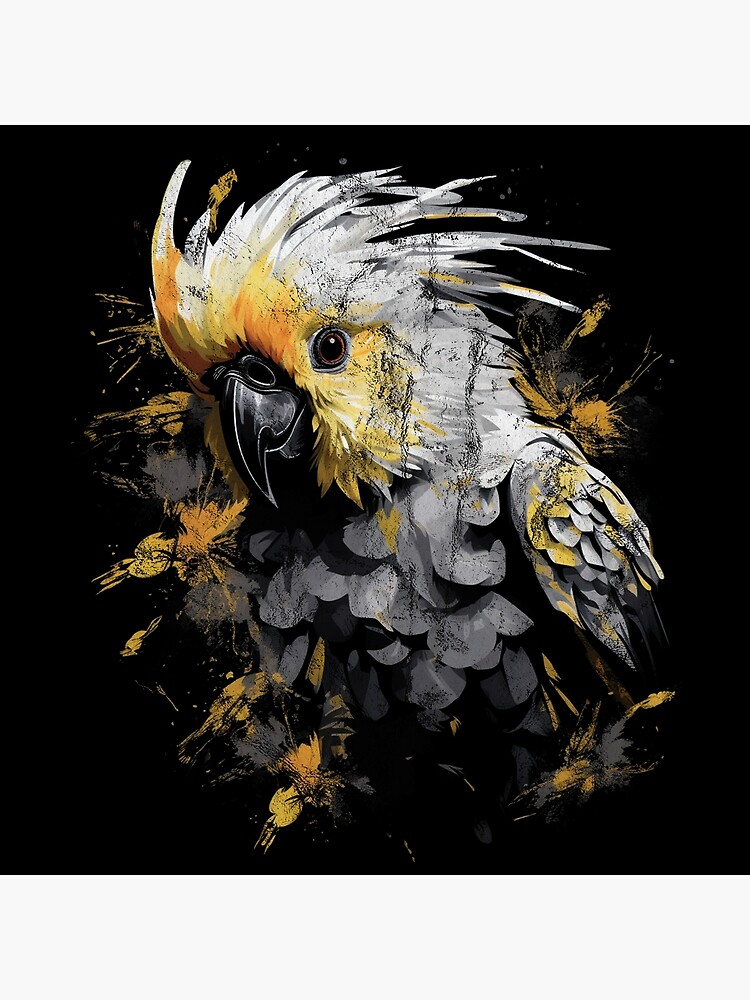This artwork, possibly AI-generated, features a striking, detailed depiction of a bird resembling a cockatoo or parrot. The bird has a prominent black beak with two large nostrils at the top, accented by yellow and orange hues around the beak and brown-ringed eye. Its head is adorned with slicked-back white and gray feathers, and a mix of gray splotches covers the chest. There is one wing visible on the right side, comprising white, gray, and yellow feathers. The bird appears to dissolve into abstract splashes of yellow and orange paint as it extends away from the detailed head and chest. The entire scene is set against a pitch-black background, enhancing the contrast and boldness of the bird's form.